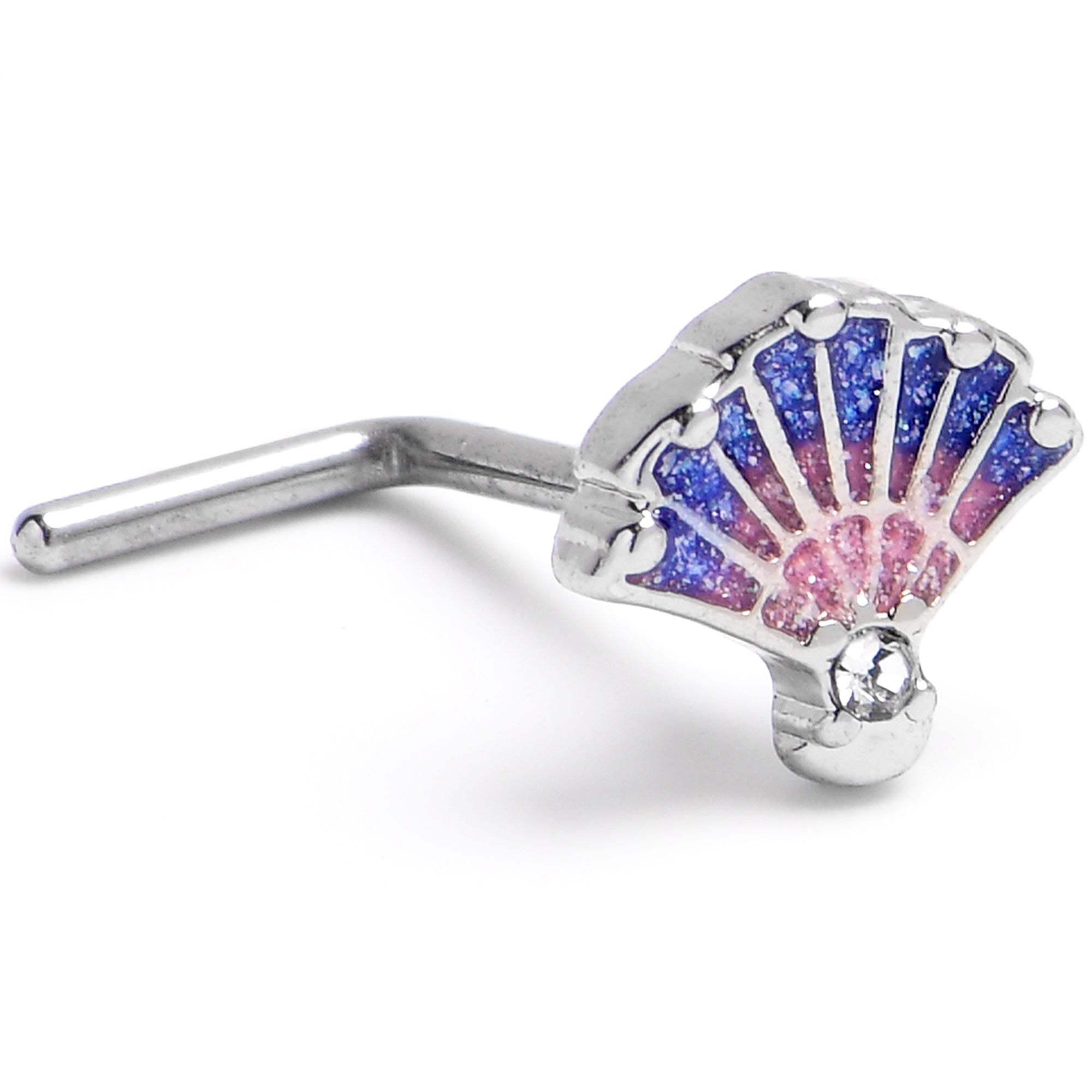This detailed close-up photograph captures an intricate piece of jewelry designed to resemble a handheld fan or a bivalve shell. The fan-like structure is outlined in silver, with a scalloped, wavy-edged exterior that adds a touch of elegance. The fan is divided into sections by silver lines, each concluding in tiny circles, except for every alternate line, which ends seamlessly at the outline. 

The inner layers of the fan start with a light lavender or pink section closest to the silver handle, that has a cubic zirconia or diamond at the base shimmering brilliantly. Moving outward, the colors transition from lavender to a rich, sparkling blue, creating a gradient effect that enhances its visual appeal. 

The fan handle, which extends from the back, bends at a 90-degree angle, forming an L-shape that suggests it might be part of a cufflink, brooch, or earring, though it’s unclear exactly how it affixes. The meticulous craftsmanship and multicolored, gem-esque appearance add to its allure, making this piece both unique and eye-catching.